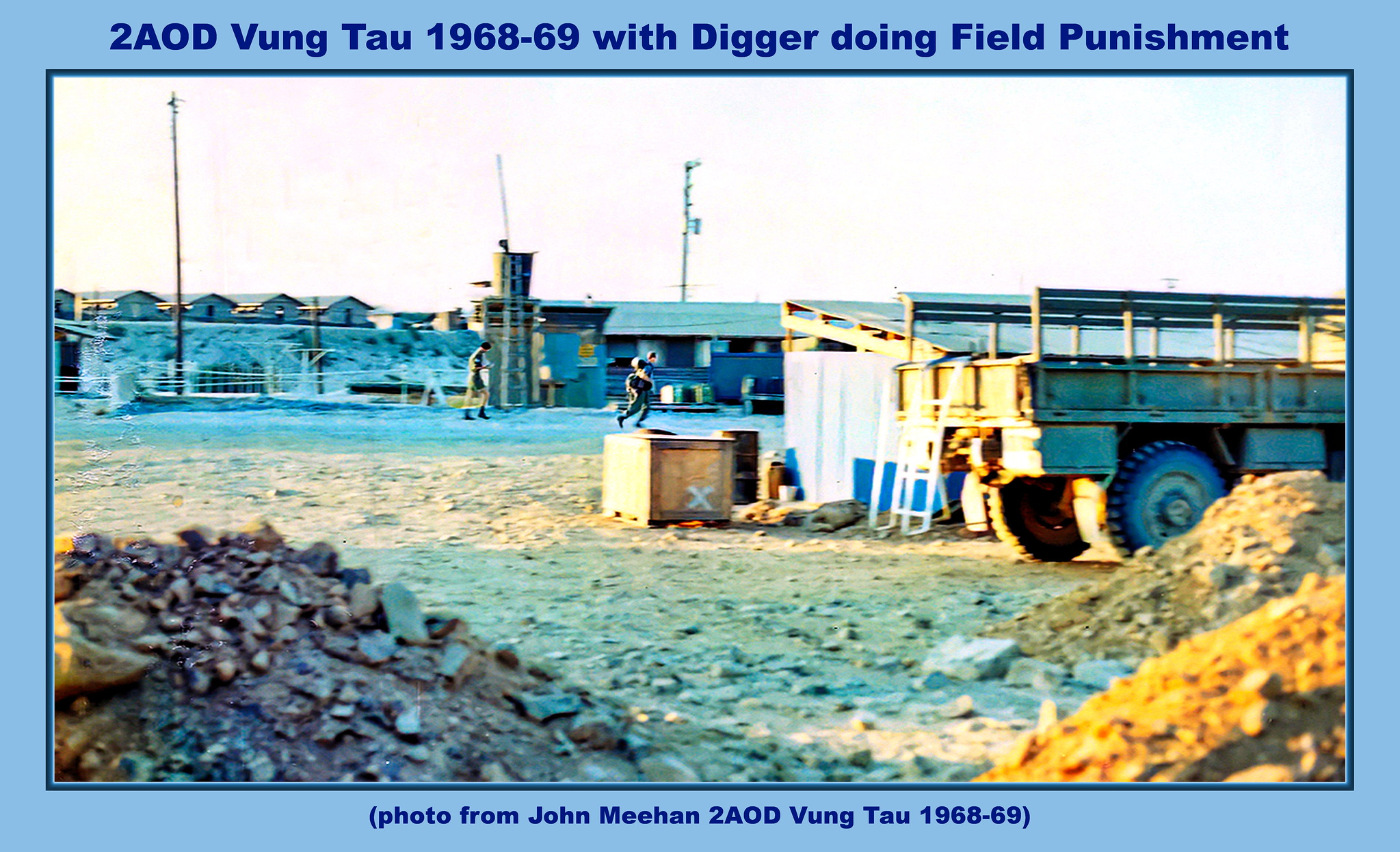The image is a landscape-mode photograph framed with a periwinkle blue border that features a darker blue pinstripe around the edges. At the top of the border, bold dark blue text reads "2AOD VUNG TAU 1968-1969 WITH DIGGER DOING FIELD PUNISHMENT." In the center bottom of the border, there is smaller, dark blue text in parentheses that notes, "Photo from John Meehan 2AOD Vung Tau 1968-1969." 

The photograph depicts a construction site or rock quarry with a foreground filled with large, chunky piles of dirt and rocks. On the right side and slightly in the middle ground, a big utility truck is visible, positioned next to some boxes and crates. In the far distance, a row of small buildings can be seen, along with a few construction workers or people running across the quarry field. The upper half of the image is dominated by a light gray sky, contributing to the overall desolate ambiance of the scene.